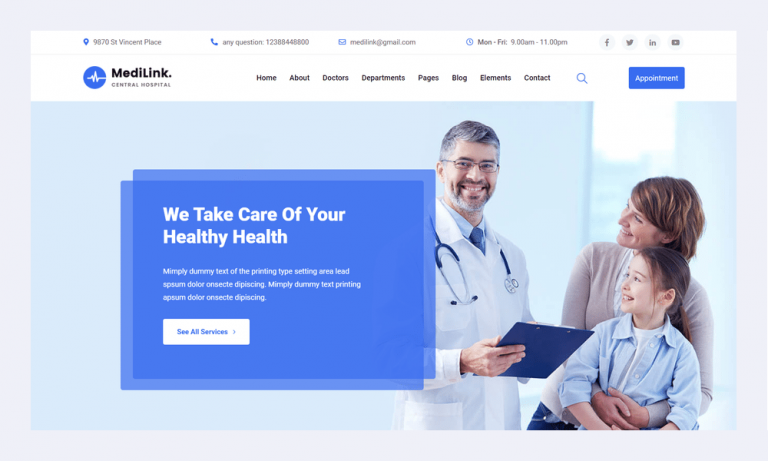The image showcases the homepage of Medi-Link Central Hospital. The top portion of the page is white, featuring the hospital’s address (9870 St. Vincent Place), contact information (Phone: 123-884-4880, Email: medilink@gmail.com), operating hours (Monday through Friday, 9 a.m. to 11 p.m.), and social media links (Facebook, Twitter, LinkedIn, and YouTube). 

Centered prominently is the Medi-Link logo with a navigation bar alongside it, including links labeled Home, About, Doctors, Departments, Pages, Blog, Element, and Contacts, plus a search icon. A blue button labeled "Appointments" sits conspicuously in white text. 

Below the navigation bar, a large photograph dominates the page. The image features a male doctor in a white coat with a stethoscope around his neck, wearing a blue tie, blue shirt, and glasses. He has short black and gray hair, a matching beard and mustache, and a pale complexion. He is smiling warmly at a woman and a young girl standing beside him. The woman, who has red-brown hair, is holding the girl around her torso. Both the woman and the girl, who has darker red-brown hair, are looking at the doctor and smiling. The overall impression is one of trust and comfort within the hospital setting. A blue rectangular banner overlaps this photograph horizontally, though its text content is not visible.